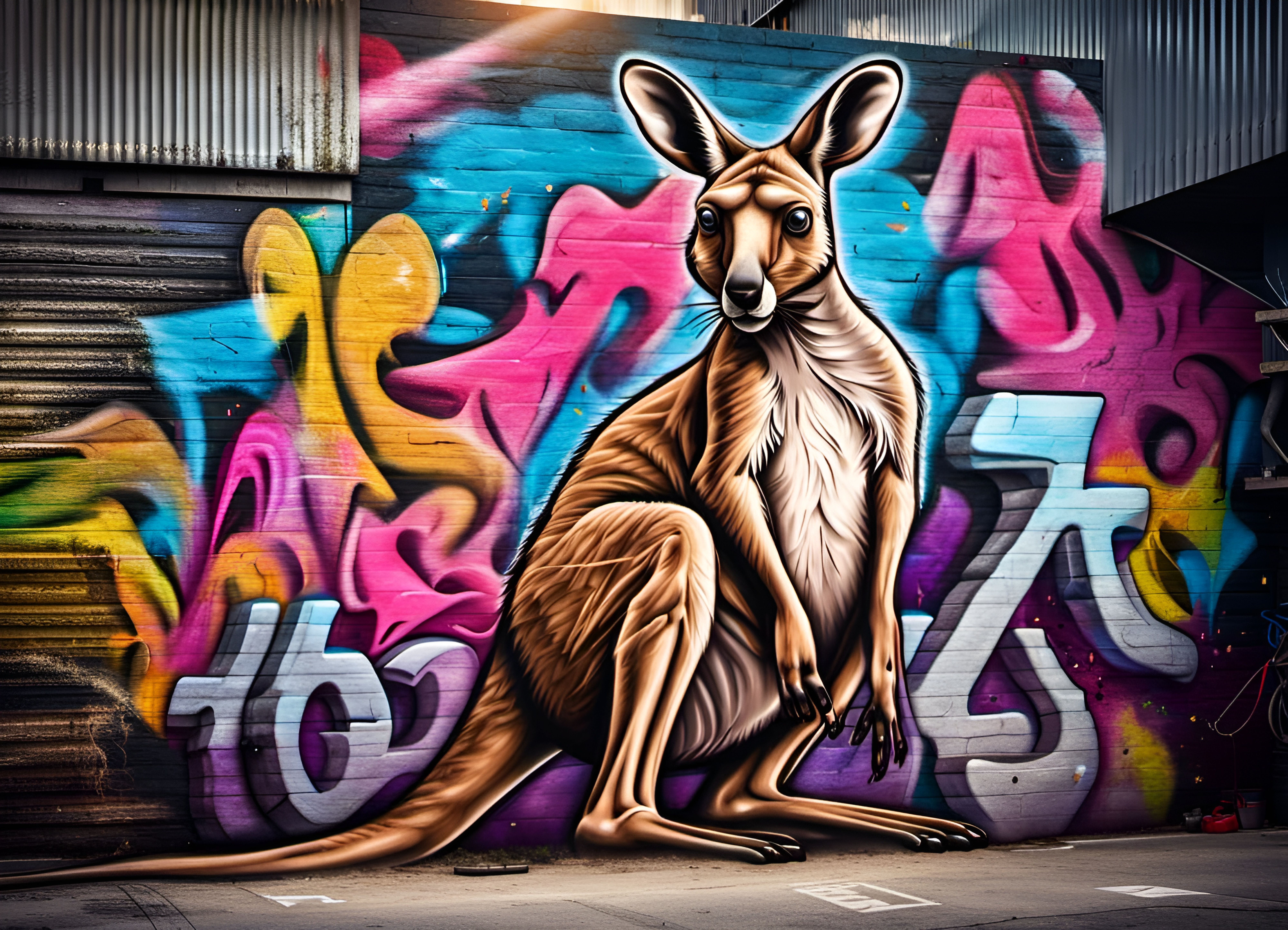The image depicts a vibrant and detailed spray-paint graffiti mural on the side of an industrial building with a black-painted brick wall and corrugated metal elements. Dominating the center of the composition is a large, light brown kangaroo with a white chest and snout, big black eyes, a black nose, and large straight ears. The kangaroo's powerful legs and gigantic feet are depicted prominently, with its smaller forearms hanging down. It is positioned against a background filled with intricate, colorful gradients of pink, yellow, blue, and purple, giving a smoky effect. Surrounding the kangaroo are scattered white block letters, including T, B, Z, J, and T, that do not form any coherent words. This dynamic and eye-catching artwork brings a splash of color and character to what appears to be a gray sidewalk in an industrial area.